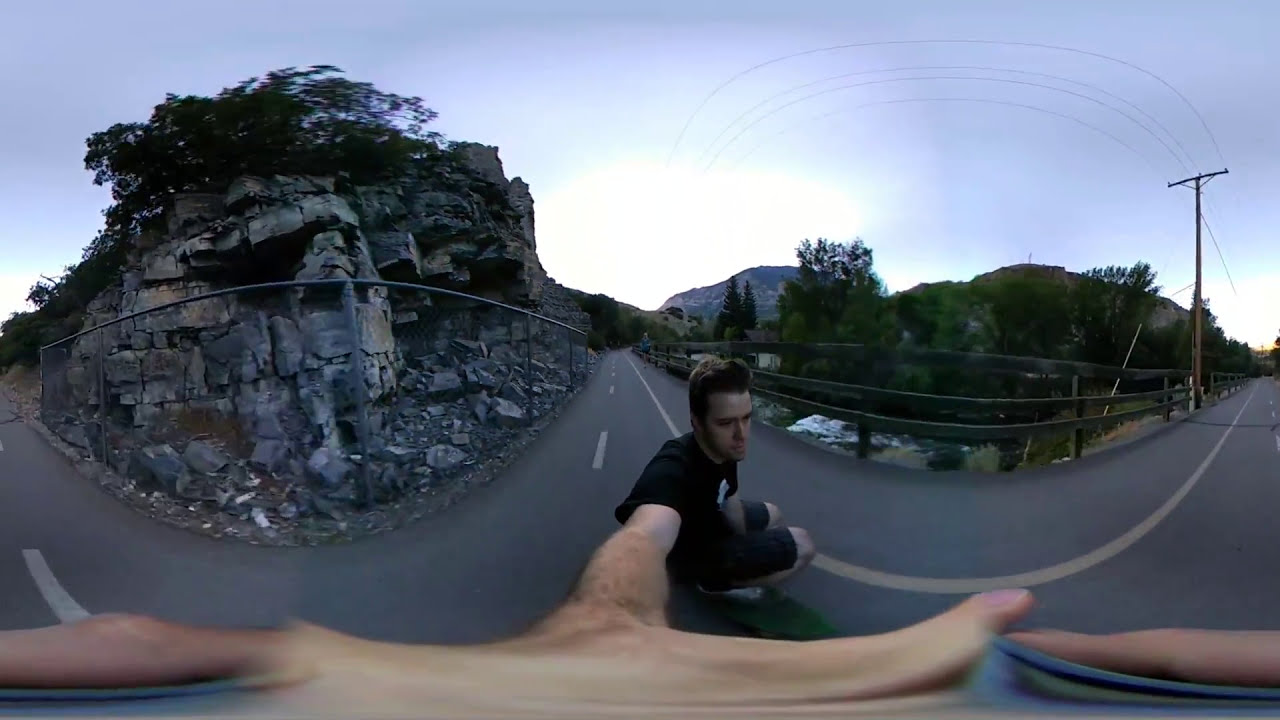The image is a warp-distorted, panoramic 360-degree photograph showing a young man squatting in the middle of a W-shaped street, with his hand stretched out and holding a camera, creating an elongated arm effect that nearly covers the entire front of the picture. He has dark hair, styled with a slight bouffant in front, and is dressed in a black hoodie, dark t-shirt, and dark shorts. His skateboard, a green one, lies on the road beside him. The street, which normally appears straight, has been warped to bow towards the viewer, creating a visually striking distortion. 

To the left of the scene, there is a rocky hill with a rock formation where slabs of rock appear to be falling off, necessitating a protective fence at the bottom. Trees cover the top of this formation. On the right, a wooden fence runs alongside a wooded area with some greenery and potentially a stream beneath, indicated by visible water. A telephone pole is also visible in this area. The sky above is a light to medium blue, dotted with white clouds, framing the surreal and warped landscape.